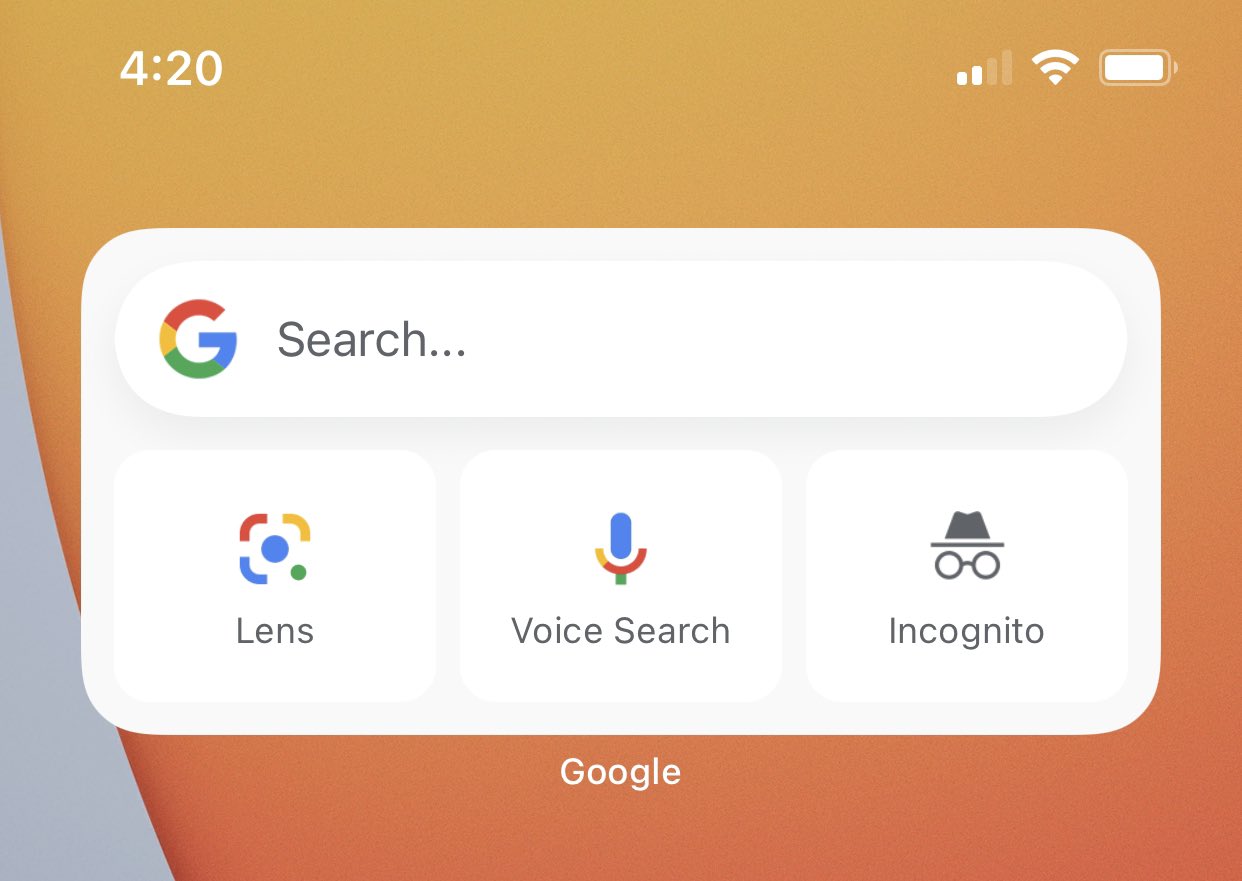The image depicts a widget likely from an Apple product, possibly an iPhone. At the top of the screenshot, the time is displayed as 4:20, accompanied by indicators for cellular data, Wi-Fi, and battery level on the right. The central focus of the image is a Google widget. This widget features a prominent search bar at the top, along with three distinct buttons beneath it: 'Lens' on the left, 'Voice Search' in the center, and 'Incognito' on the right. The overall layout and design elements strongly suggest that the widget is designed for quick and easy access to essential Google functionalities.